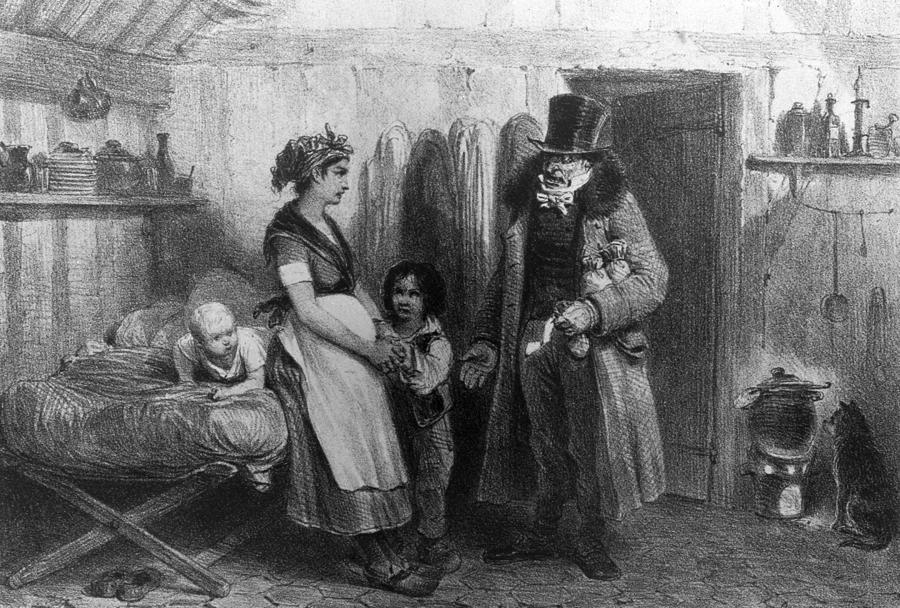This intricately detailed black-and-white sketch, likely from the 19th or very early 20th century, depicts the austere interior of a Paris slum. At the center of the scene, a possibly pregnant woman, wearing a simple long dress and a white apron with her hair wrapped in a cloth, leans against a bed cradling an infant. To her right, a small boy holds her hand, supporting her. The setting reveals a modest living space with a portable furnace in one corner, next to which a dog is seated.

A man, characterized by his tall, shiny top hat and fur-lined trench coat, stands authoritatively to the left of the dog, near a doorway. He appears stern, holding a piece of paper, possibly an eviction notice or a bill, and his expression is serious, almost angry. His presence suggests he might be the landlord of this humble abode. The room contains sparse furnishings, including a cot on which the baby is seated, shelves holding simple items like candles and plates, and utensils hanging against the wall. The sketch's fine lines and detailed shading provide a vivid portrayal of the harsh living conditions of the time, with walls that appear worn and stone floors that add to the overall gritty atmosphere.